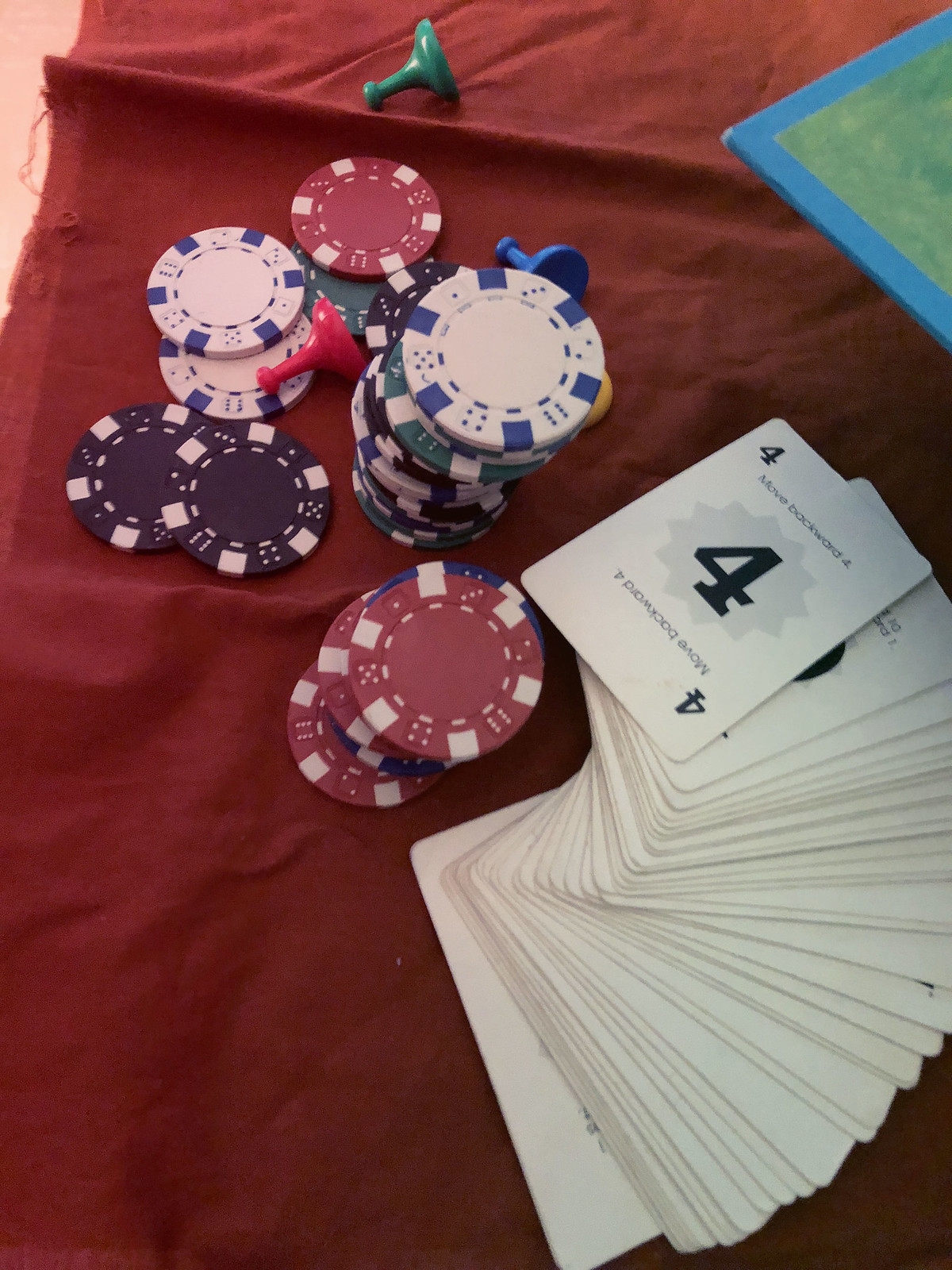In this photograph, we see a gaming setup on a vibrant red sheet, with a hint of a pink background on the left side, suggesting a pink floor. On the right side, partially cut off, is the inside of a game board box, adding context to the scene. Dominating the foreground is a fan-shaped spread of cards, the topmost displaying the number four within a starburst design and indistinct writing, indicating these are not standard playing cards. Adjacent to the cards are multiple stacks of poker chips. The stack in the center features a red chip on top with white markings, accompanied by a taller stack with a white chip on top and another stack with a red chip. Further left, you notice a standalone white chip, and in the very front on the left, two dark blue chips are evident. Scattered among these chips are colorful player pieces—a green, a red, and a blue—situated on what appears to be a game board, hinting at a game in progress or about to commence.